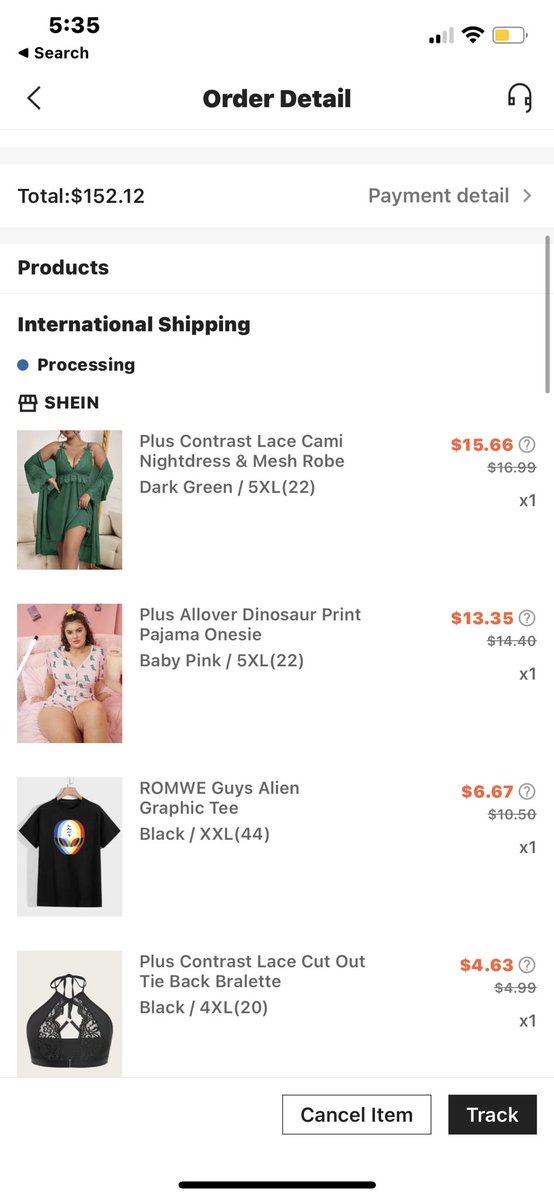The screenshot captures a mobile shopping interface on a user’s cell phone, set against an all-white background. In the top-left corner, the time displays as “5:35” in black. Directly below, the word “Search” accompanies a left-pointing arrow. On the right side of the screen, a battery icon is half yellow and half white, next to a fully black Wi-Fi symbol. The internet signal icon is half black and half gray, and a gray van symbol points left in the center of a black-bordered detail.

Further down, a headphones icon appears just above a light gray border. To the left, against a white background, "Total: $152.12" is written in black, while on the right, “Payment Detail” is also in black next to another gray border. Below these elements, "Products" is bolded in black and followed by "International Shipping." A blue dot indicating “Processing” is situated below.

On the right, a thin gray vertical bar runs down the side. Further below, a shopping icon labeled “SHEIN” appears on the right. Under this, there are sequential images of various items: a woman in a green dress, a girl in a white polka dot bikini, a black shirt, and a black bra. To the right of each image, the product’s name and its color are listed, with the price displayed in red underneath, followed by another price in black. Each item is marked with a quantity of “x1” in the shopping cart.

In the bottom right corner, a black tab with “Track” in white letters is visible. To its left, a white tab with a black border displays the option “Cancel Item.” Central toward the bottom, a black border spans roughly an inch on either side.